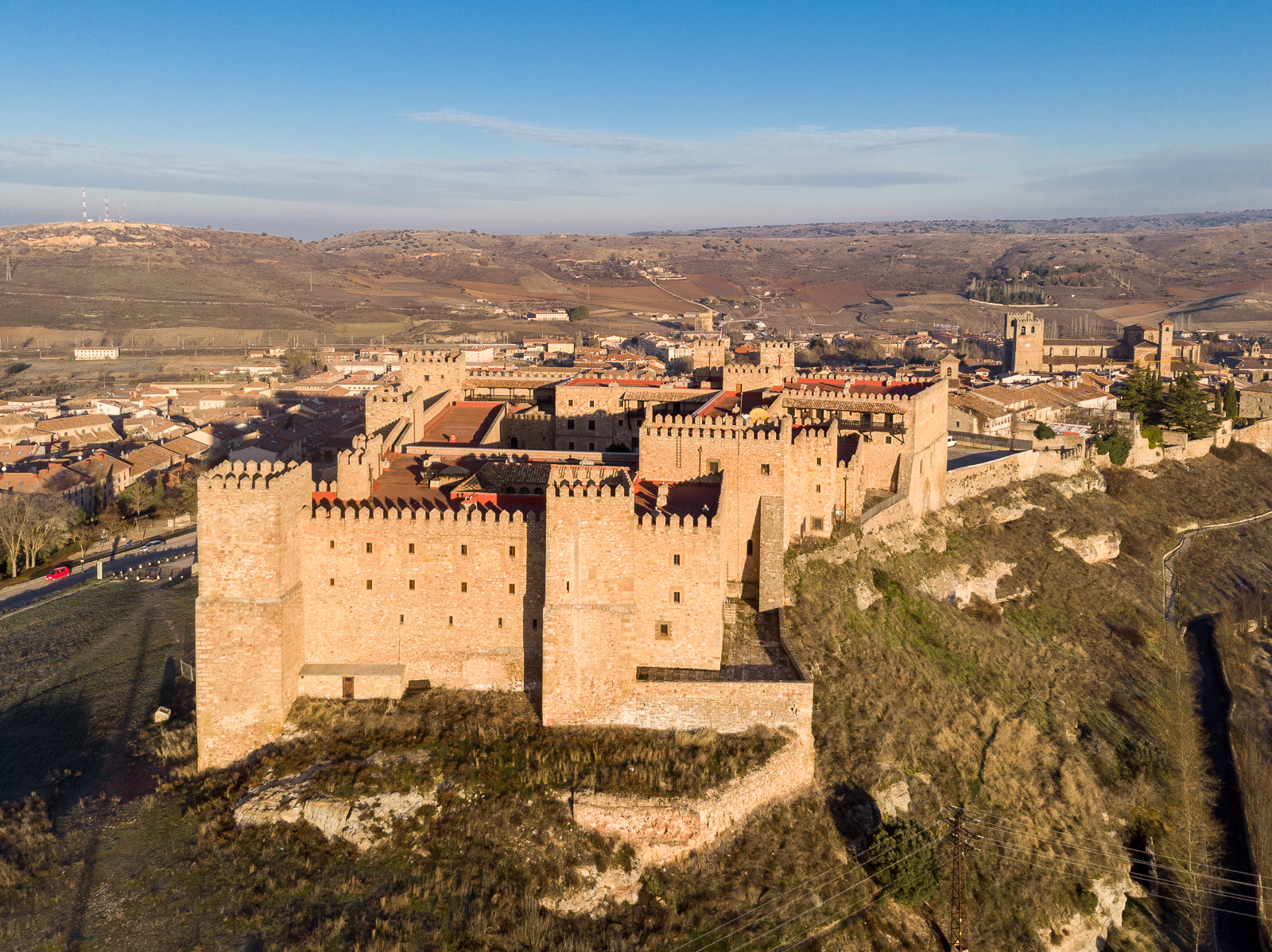This is an angled aerial photograph of an expansive, historic castle, likely from the medieval era, possibly situated in England or a similar region. The castle, constructed from beige stone or brick, is perched dramatically atop a greenish rocky hill and bordered by steep cliffs on the edges. The imposing structure features at least ten towers, giving it a fortress-like appearance. It reaches approximately five to six stories high and exhibits a somewhat rectangular layout with multiple sections and square corner towers adorned with ramparts. 

Inside the castle walls, several buildings with orange-colored roofs are visible, along with a sturdy stone fence surrounding the main keep. A road on the left and a walking path on the right suggest access points to the castle, which stands prominently near the edge of a cliff. Beyond the castle, a small town can be seen, with hills and a clear blue sky forming the picturesque background. The landscape around the castle includes mostly brownish land with sparse vegetation, enhancing the fortress's formidable and historic presence.